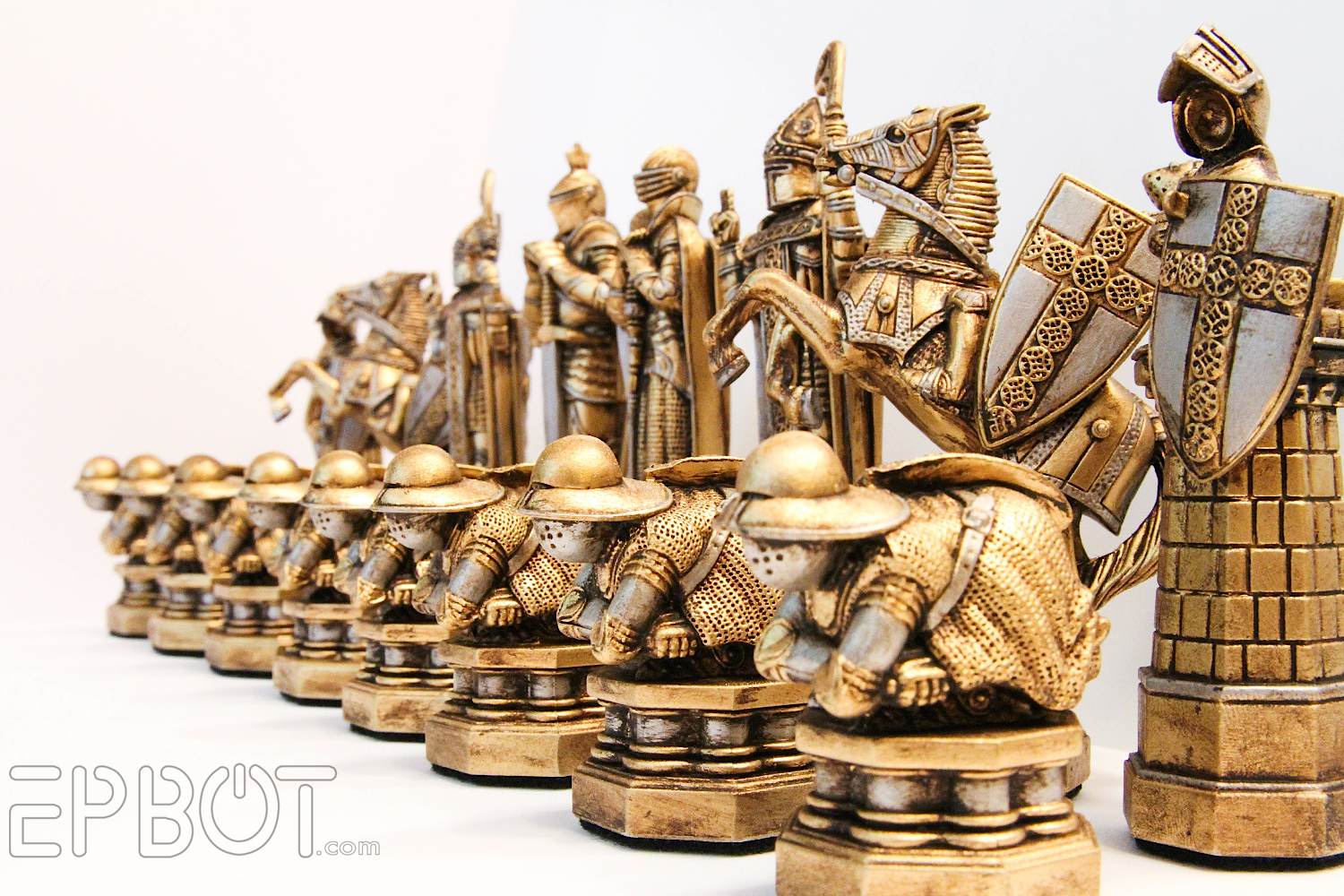The image features an intricate chess set, seemingly sourced from EPBOT.com, showcasing a half-view of the board. Dominating the right-hand side of the picture and angling upwards toward the left, the set includes both large and small pieces, all cast in a striking gold hue. The foreground features several identical pawns, each resembling a bent-over figure kneeling on pedestals with helmets, gloves, and capes, almost like turtles with arms. In the background, more prominent figures represent knights and rooks. The knights, depicted as big, shield-bearing warriors, stand alongside a rearing horse. The rooks are designed with castle-like bases made up of irregularly shaped bricks. The entire arrangement sits on a disc or platform, with the text "EPBOT.com" visible in a stylized font at the bottom left of the image. The detailed craftsmanship gives an impression of a grand, historic battle scene captured in gold.